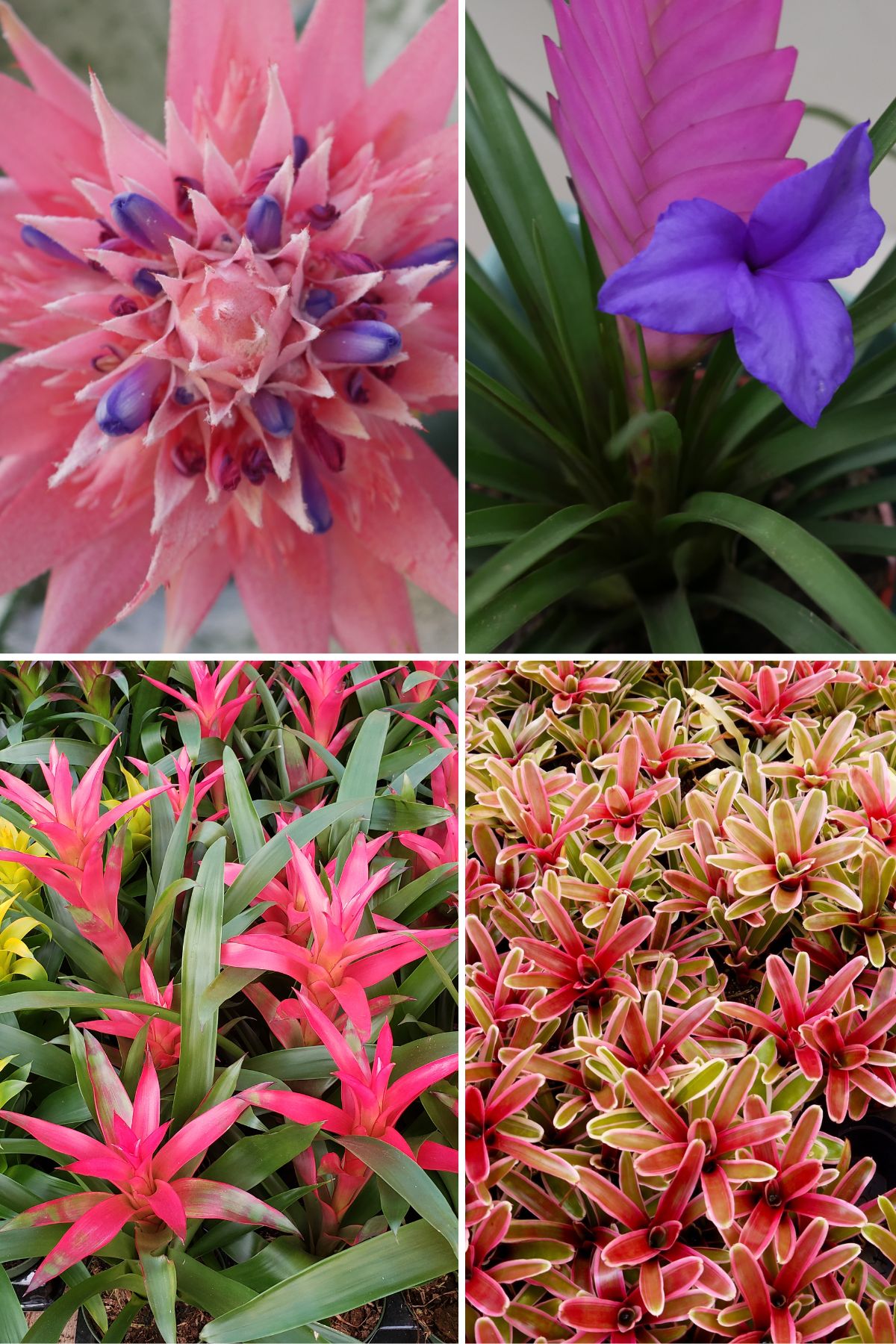The image comprises a 2x2 grid of four close-up photographs of various vibrant flowers. Each picture showcases a distinct type of flower, highlighting their unique characteristics and vivid colors. In the top left, there is a striking pink flower with spiky petals. The top right features a purple and pink flower with three prominent petals and large green leaves. The bottom left displays a collection of pink flowers encircled by long, green foliage. The bottom right shows flowers with both pink and green hues, characterized by their rounded petals. Taken outdoors during the daytime, these zoomed-in images reveal intricate details and a stunning array of colors, including green, light pink, pink, light yellow, violet, dark green, and fuchsia, with subtle hints of yellow.